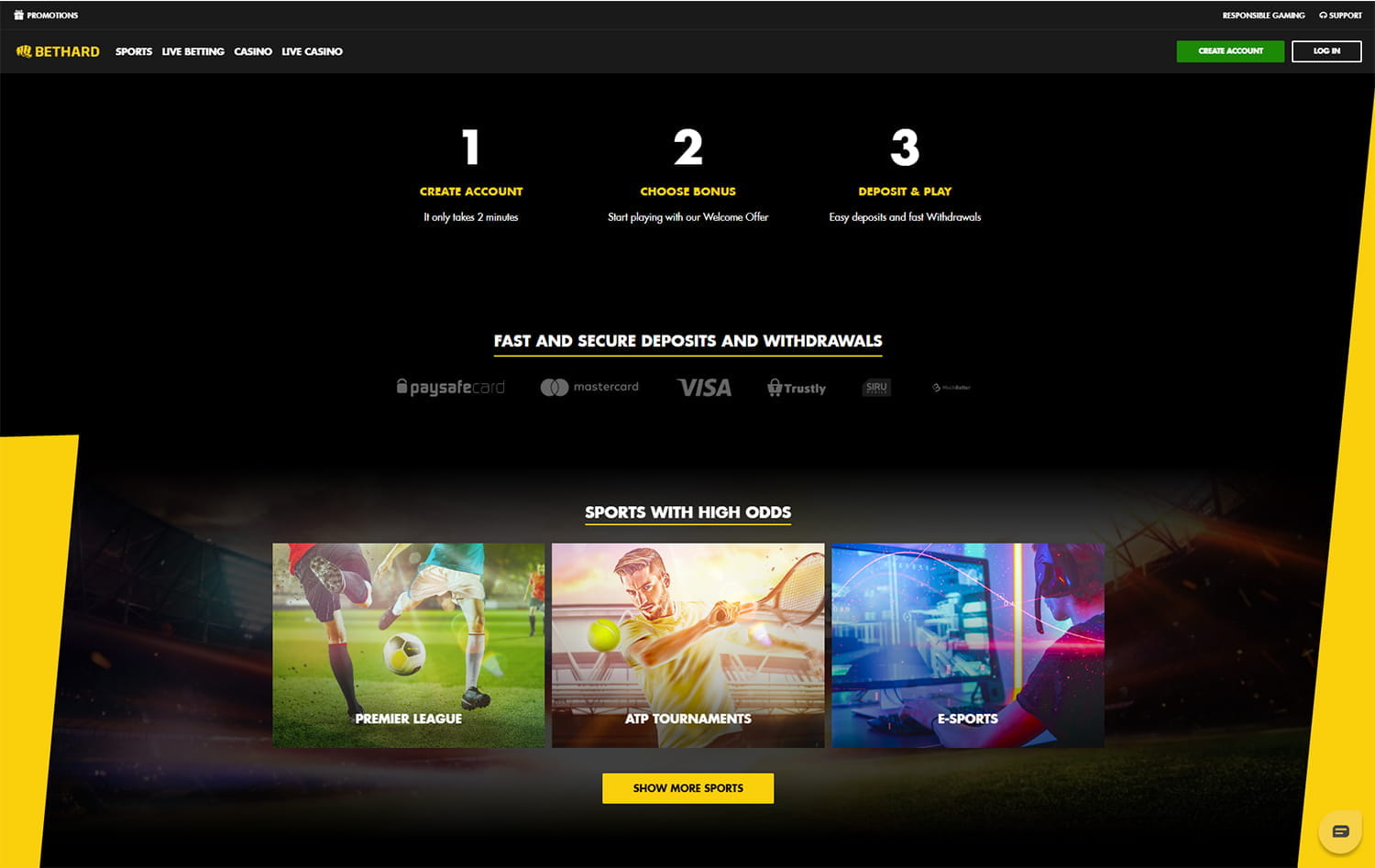The image is a detailed screenshot from a computer screen displaying a sports betting website. In the top left corner, the word "Promotions" is prominently shown in white font. On the top right, there are buttons labeled "Responsible Gaming" and "Support." Along the top taskbar, on the left-hand side, the labels "Bethard," "Sports," "Live Betting," "Casino," and "Live Casino" are listed consecutively. To the right, a green button saying "Create Account" is displayed, with the text in white, alongside a "Login" button.

Beneath these elements, the process to get started on the website is outlined in three steps: 1) "Create Account. It only takes two minutes," 2) "Choose Bonus. We're playing with our welcome offer," and 3) "Deposit and Play. Easy Deposits and Fast Withdrawals." This section is followed by the message "Fast and Secure Deposits and Withdrawals," supported by logos for Paysafe, MasterCard, Visa, and Trustly.

Below this informational section, three promotional images are displayed: 
1. On the left, it reads "Sports with High Odds - Premier League," accompanied by an image of soccer players in action.
2. In the middle, the text "ATP Tournaments" appears with an image of a tennis player holding a racket.
3. On the right, "eSports" is displayed along with an image of a person wearing a headset in front of a computer screen.

Finally, at the bottom, there is a button labeled "Show More Sports" inviting users to explore additional sports options.